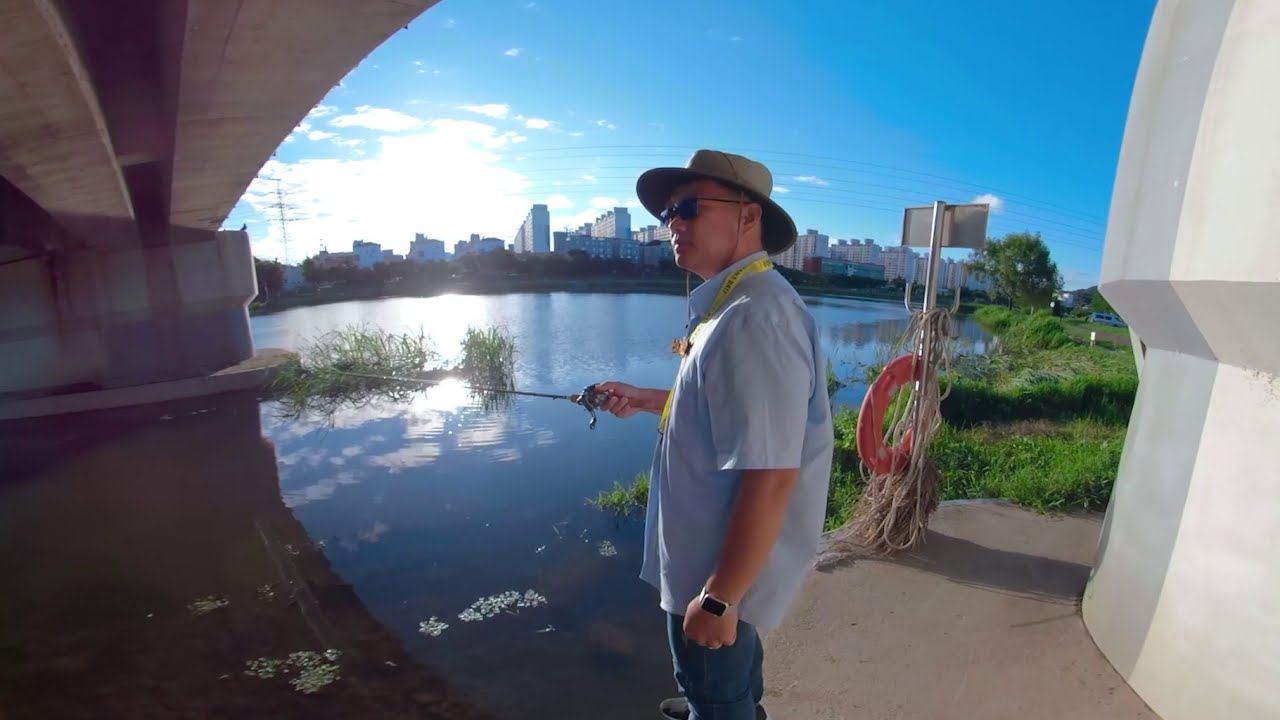The photograph captures a man fishing in a shallow waterway partially sheltered by the concrete framework of a bridge or freeway. He is positioned centrally, facing left, with his right hand holding a fishing rod extended into the water. The man is dressed in a light blue short-sleeve button-up shirt, blue jeans, a tan fisherman's hat reminiscent of Indiana Jones, sunglasses, a yellow lanyard around his neck, and a watch that looks like an Apple Watch. 

On the right side of the image, a silver metal pole with an obscured sign has a life preserver and some rope wrapped around it. The pole marks the beginning of a curving sidewalk that transitions into a grassy area. Beyond the sidewalk, there is more grassland and scattered shrubs, some of which are also visible in the water, suggesting the water's shallowness. The water has a somewhat murky appearance with greenery growing on its surface.

To the left, the base of the bridge is visible, and its support structure offers a stark contrast to the open, bright blue sky seen further out in the background. Above the man's head, a city skyline filled with various buildings stretches across the horizon, under the clear blue sky that contains a few clouds and suggests bright sunlight reflecting off the water.